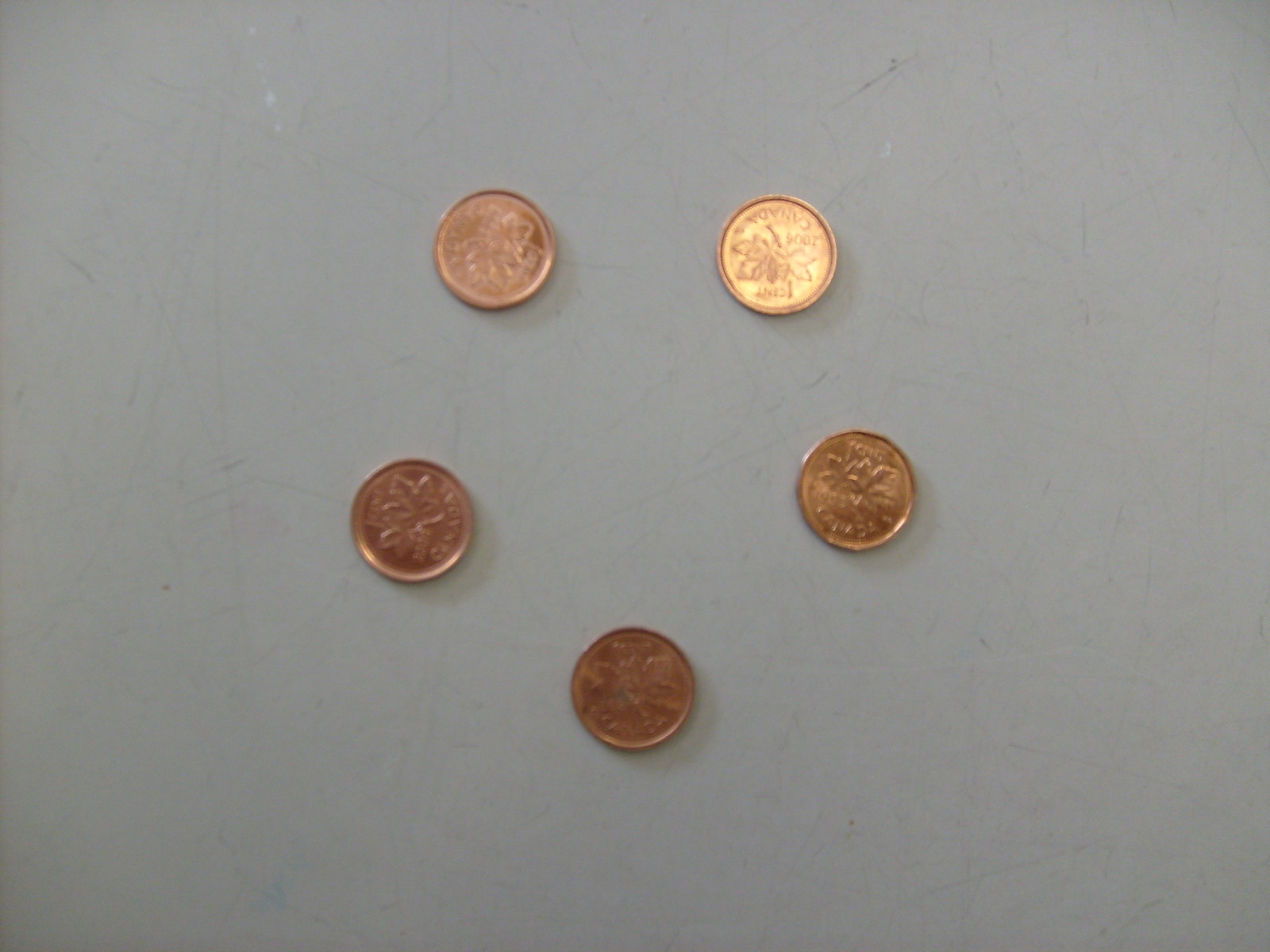This photograph features a light gray surface that appears to have thin, barely noticeable black scratch marks or pencil scribbles. Arranged on this surface are five Canadian copper pennies, forming an upside-down pentagon shape. Each penny displays the image of a maple leaf in the center, with "Canada" inscribed below. The pennies vary in appearance, showcasing different degrees of aging, from shiny and reflective to dark and tarnished. The penny positioned in the upper right corner is particularly illuminated by a light source from behind the camera, highlighting the variations in their luster and coloration.